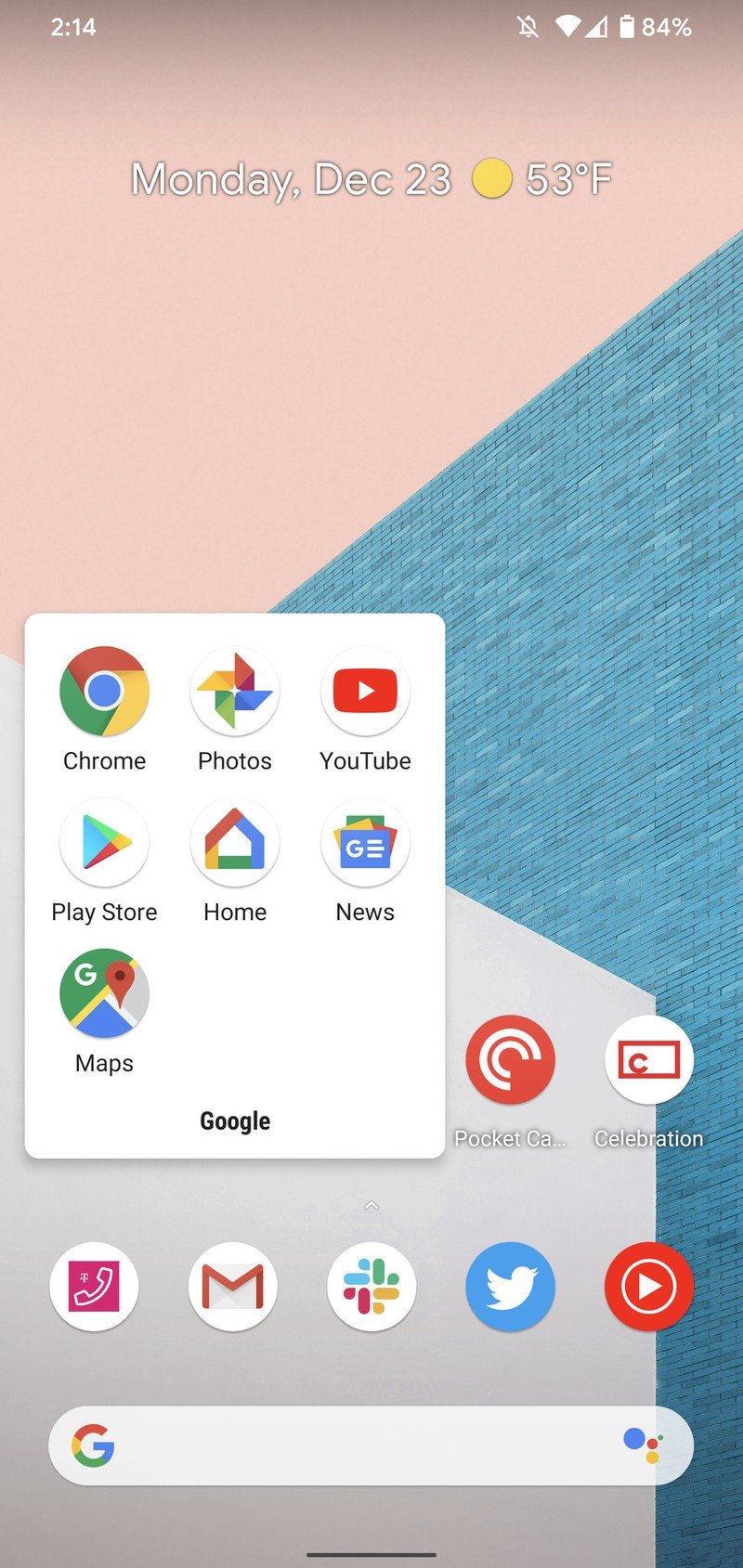This image appears to be a screenshot of a tablet or smartphone displaying its home screen. In the top left corner, the time is shown as 2:14, accompanied by Wi-Fi symbols and an 84% battery level indicator. At the top center, there's a weather widget indicating the location is Texas, with the date Monday, December 23rd, and the temperature at 53 degrees Fahrenheit, symbolized by a sun icon.

Prominently displayed in the middle of the screen is a white box containing multiple app icons, including Chrome, Photos, YouTube, Play Store, Home, News, and Maps. To the right of these icons, there are additional ones labeled Pocket and Celebration. Beneath these, you can see more app icons: a telephone, a Google Mail icon (commonly identified as an 'M'), a colorful icon, a Twitter icon, and a red music play button icon.

Further down, there is a white Google search bar, and at the very bottom of the screen, there's a black line spanning the width of the screen. The background features a design with colors like peach, gray, and blue, forming an abstract pattern.

This setup strongly suggests that the screenshot is from an Android device's home screen, particularly showcasing several Google-related apps and icons.